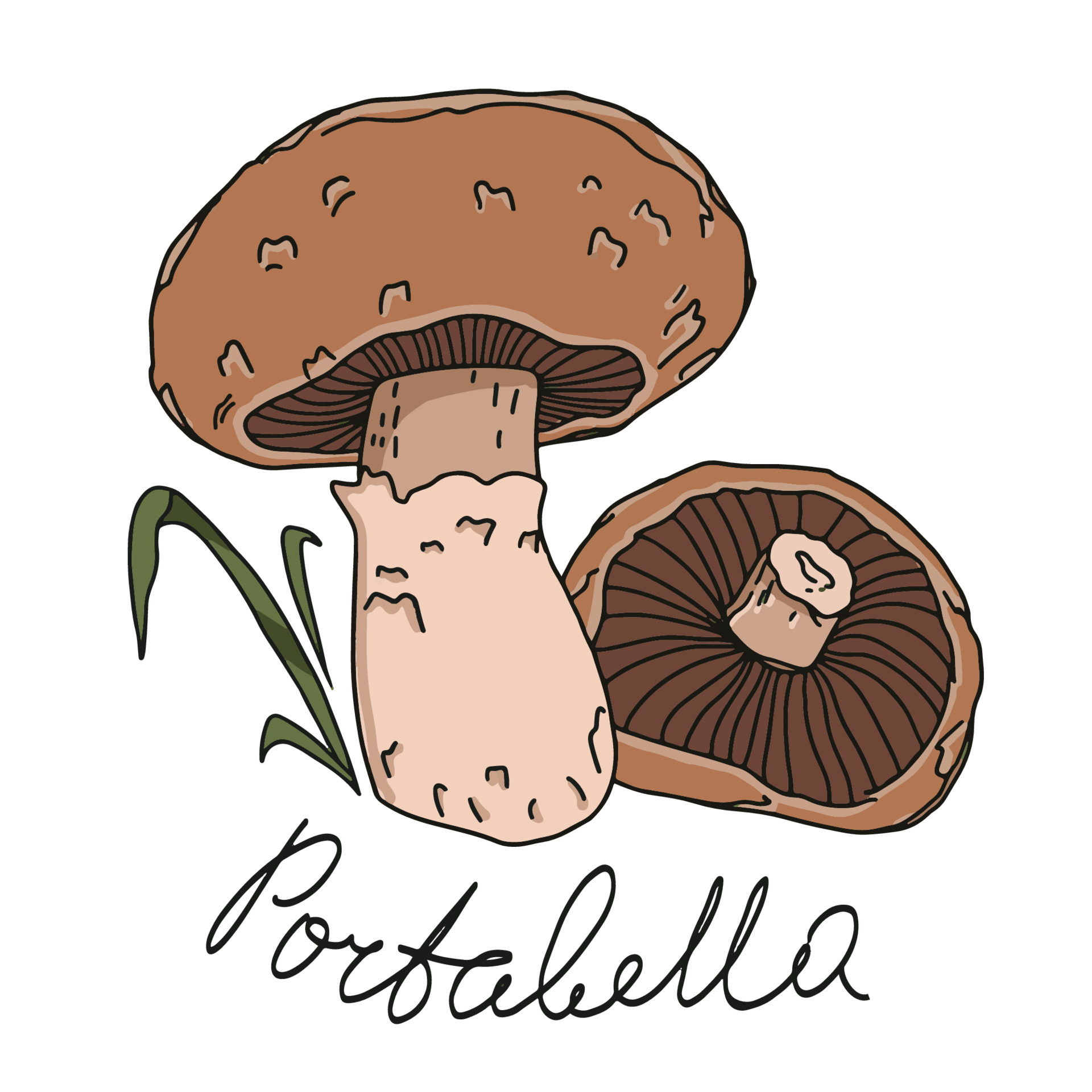In this detailed illustration, we see two portobello mushrooms prominently displayed with the word "portobello" written in elegant black cursive at the bottom. The primary mushroom stands upright in the center, featuring a grayish stem with subtle black specks and a large, dark brown cap. A pinkish-purple hue adorns its underside. Next to this mushroom, three blades of green grass extend from the left side of its stem, providing a touch of natural detail.

Beside the standing mushroom lies another mushroom, which is overturned with its severed stem exposed. The top cap, now facing the ground, shares the same dark brown color as the first mushroom, while its underside reveals dark brown ribs radiating from the center with lighter brown edges. This underbelly is richly detailed, showing intricate ridges and black markings that stretch from the stem to the outer portions of the cap. Both mushrooms exhibit a harmonious color scheme of varying browns and intricate textures, lending a realistic and earthy feel to the illustration.